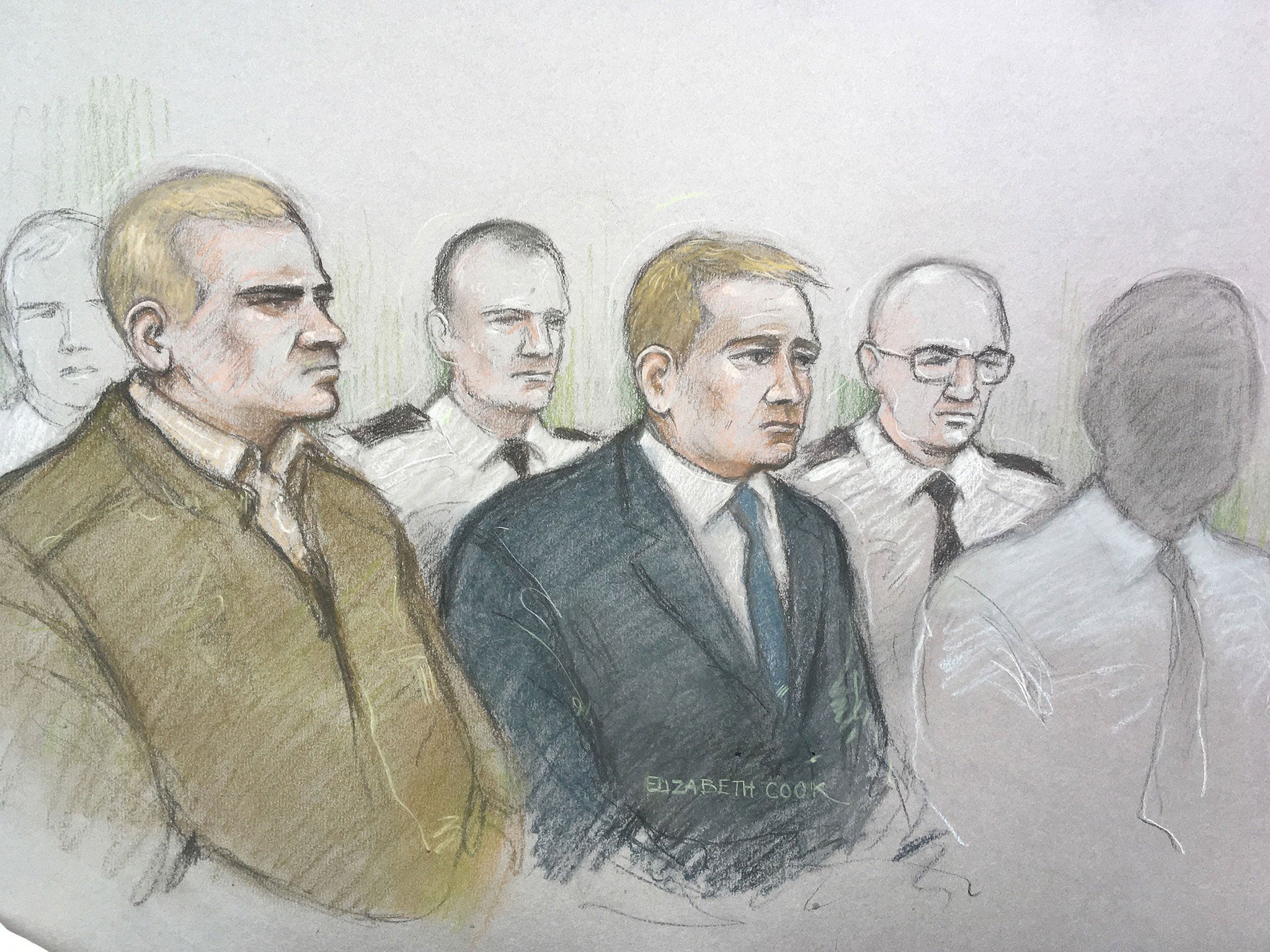This image appears to be a detailed, colored drawing or courtroom sketch on a textured light gray paper, possibly using charcoal or colored pencils. Central in the sketch, there is a man in his 30s or 40s, with short blonde hair, wearing a navy or black suit, a white shirt, and a blue tie. He is facing slightly to the right with a neutral expression. To his left is another white man with brownish hair, dressed in a light brown or mustard-colored zip-up jacket and a white shirt. This man, also facing to the right, has a similar smirk to the man in the suit.

To the right of the central figure, there is a man whose face is grayed out, wearing a white shirt and a gray tie. Further to the right, there is a court officer, a white man with glasses, a white shirt, black tie, and black epaulets, looking mostly forward. Behind this court officer, another younger, balding officer without glasses, also in a similar uniform, is positioned. 

Behind the man in the brown jacket, there is a faintly drawn male face in the upper left-hand corner. The backdrop of the scene is also gray. Across the body of the central figure, the text "Elizabeth Cook" is watermarked.